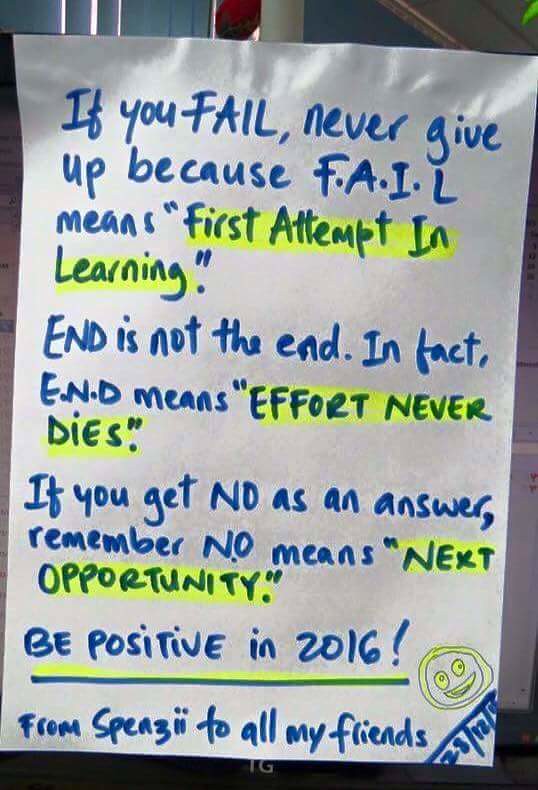The image features a sheet of paper that occupies the center of the frame, obscuring the background. The paper, with some artifacting indicative of a low-quality photograph, appears to be taped to a surface, possibly a computer monitor, suggesting an indoor setting though it was initially thought to be outdoors. The paper contains a motivational message written in blue marker, with certain phrases highlighted in yellow.

The text on the sign reads: "If you fail, never give up because F-A-I-L means 'First Attempt in Learning.' End is not the end. In fact, E-N-D means 'Effort Never Dies.' If you get no as an answer, remember no means 'Next Opportunity.' Be positive in 2016!" The phrases 'First Attempt in Learning,' 'Effort Never Dies,' and 'Next Opportunity' are all highlighted for emphasis. Additionally, "Be positive in 2016!" is both underlined and highlighted, with a smiley face drawn next to it. At the bottom of the sheet, a personal note reads, "From Spezi to all my friends," with an unreadable date and further accented smiley face. The colors visible include blue, gray, white, red, green, yellow, black, and silver.